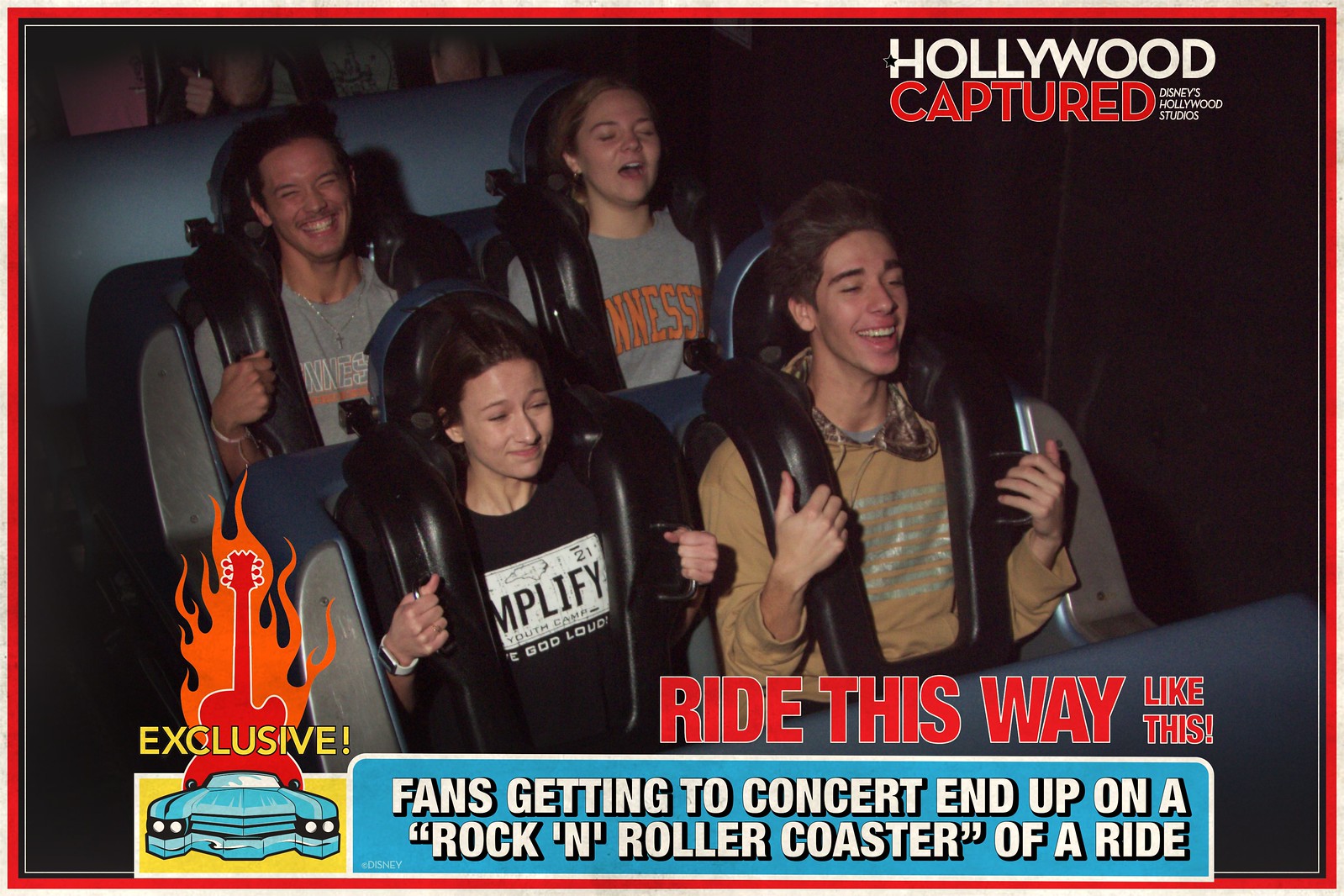This vibrant color photograph captures the exhilarating moment of four people on a roller coaster at an amusement park. The scene is centered around two rows of passengers securely fastened with black plastic seats. In the front row, a young woman on the left wears a black shirt with a white and black license plate design, while the young man on the right sports a brown sweater. Both have their eyes closed, with expressions of excitement and nerves evident on their faces. In the back row, the man on the left grins widely, clad in a gray t-shirt with white text, while the woman beside him, donning a t-shirt emblazoned with "Tennessee" in orange, has her eyes closed and mouth open in a joyful scream. 

The photograph features overlaid digital text and a red border framing the entire image. In the top right corner, it reads "Hollywood Captured" in white and red, followed by "Disney's Hollywood Studios." The bottom left corner bears the word "Exclusive" alongside an illustration of a car with a flaming red guitar on top. Dominating the bottom of the image is a large blue chyron with white text, stating, "Fans getting to concert end up on a rock and roller coaster of a ride," accompanied by red text above it proclaiming, "Ride This Way Like This." The visual elements are a lively mix of colors, including red, orange, yellow, light blue, gray, white, black, and beige, heightening the overall energetic and fun atmosphere of the scene.